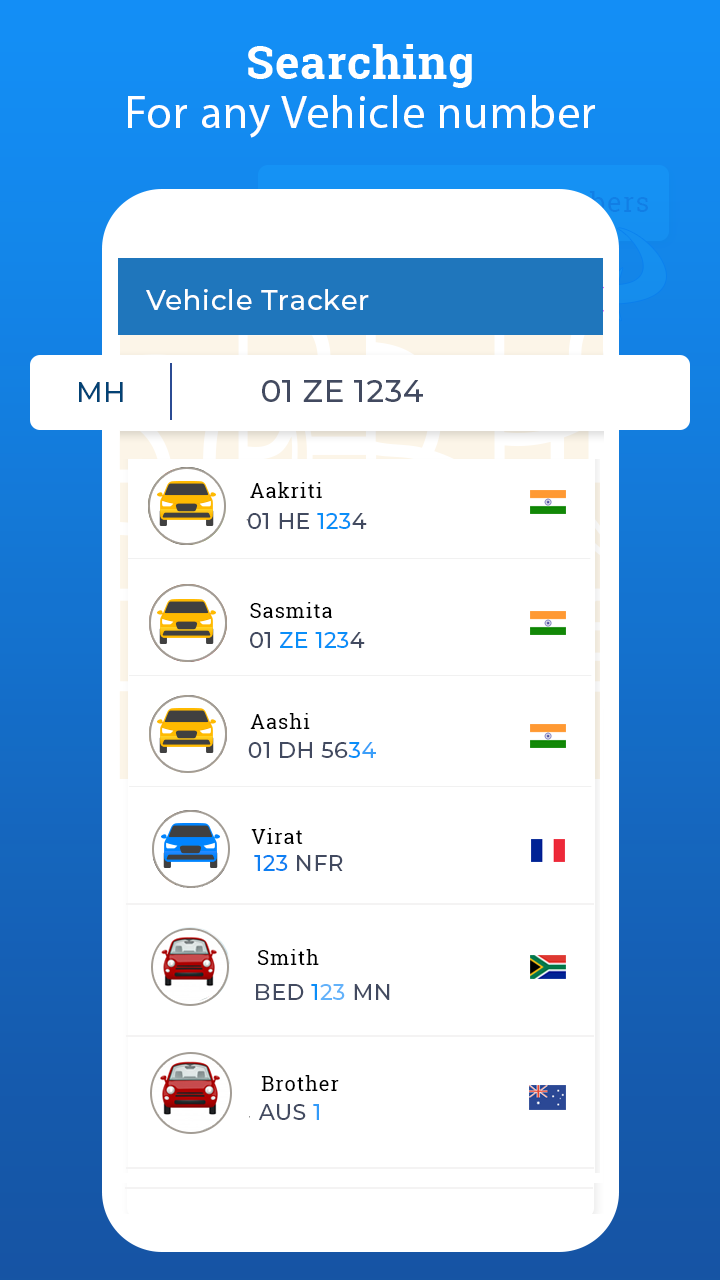The image features a background that starts with a light blue at the top and gradually transitions to a darker blue near the bottom. In the center of the top section, there is a text prompt that reads, "Searching for any vehicle number." Below this prompt is a white rectangle with rounded corners, containing a smaller blue rectangle labeled "Vehicle Tractor." Extending out from this white rectangle and intruding into the blue gradient background is another white rectangle that reads "MH," followed by a dash and the sequence "01ZE1234."

Below this, there are several circular icons with different vehicles and details:

1. A yellow car inside a black-outlined circle. Adjacent to it, there's a partial text and the sequence "01HE1234," with "01HE" in black, "123" in blue, and "4" back in black. Next to this is a flag featuring orange at the top, white in the middle, and green at the bottom with a black symbol in the center.
   
2. Another yellow car inside a black-outlined circle. Nearby, there's partial text and "01ZE1234," with "01" in black, "ZE1234" in blue, and "4" back in black. The adjacent flag is similar to the previous one.

3. A yellow car inside a white-outlined circle. The nearby text features "01DH5634," with "01DH56" in black and "34" in blue. This icon also has the same tricolor flag.

4. A blue car inside a black-outlined circle. Alongside it are partial text and "123NFR," with "123" in blue and "NFR" in black. Next to this is a flag composed of horizontal blue, white, and red stripes.

5. A red car inside a black-outlined circle. The surrounding text reads "BED123MN," with "BED" in black, "123" in blue, and "MN" back in black. The flag next to this icon features a black triangle, a green sideways Y, and red and blue sections.

6. Another red car inside a black-outlined circle. Surrounding this icon is partial text and "AUS1," with "AUS" in black and "1" in blue. This icon is accompanied by a flag that has the British flag in the upper left corner, set against a blue background with white dots.

All these graphical elements and details are meticulously arranged within the gradient blue background, providing a clear and organized layout for vehicle identification.